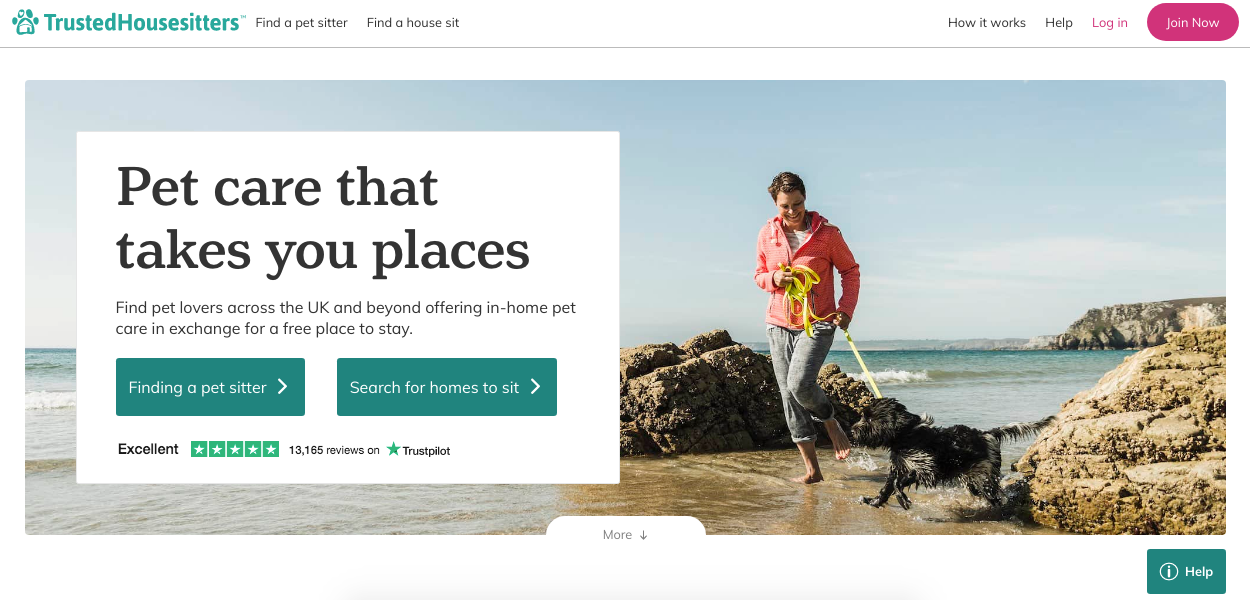This screenshot showcases the homepage of Trusted House Sitters' website. At the top of the page is the site's logo, featuring a roughly drawn house icon paired with a paw print composed of four small circles, all in green. The brand name "Trusted House Sitters" is displayed next to the logo in green letters. 

Below the logo, a menu bar in black lettering includes options such as "Find a Pet Sitter" and "Find a House Sit." On the right-hand side of the menu, it features "How It Works," "Help," and in red letters, "Log In." Adjacent to "Log In" is a prominent red button labeled "Join Now."

Centrally located on the page, the main text reads "Pet care that takes your place" in large, bold black letters. Beneath this, a subheading in smaller black letters explains, "Find pet lovers across the UK and beyond offering in-home pet care in exchange for a free place to stay."

Two rectangular green buttons are positioned below this subheading. The first button, "Find a Pet Sitter," includes a right-pointing white arrow, and the second, "Search for Homes," also features a right-pointing white arrow.

Lower on the page, in smaller yet bold black text, is the word "Excellent," followed by five green boxes each containing a white star, indicating a rating. Small digits beside this rating state "13,165 reviews on Trustpilot."